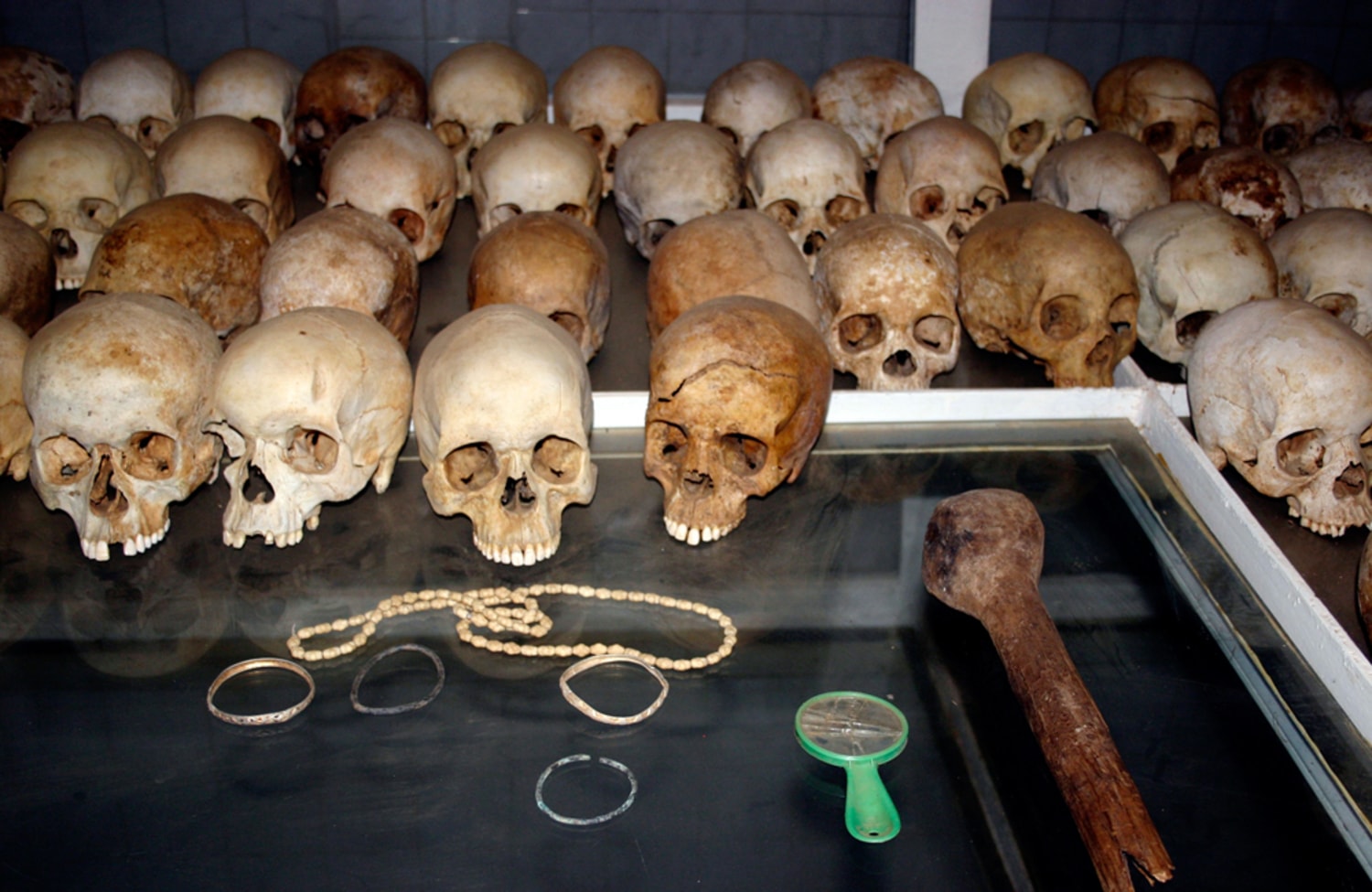This full-color indoor photograph, illuminated by artificial light, captures a staged and educational display, likely in a museum. The image, which is horizontally rectangular without a distinct border or background, prominently features three rows of human skulls arranged neatly on glass display cases. The skulls, all missing their jaws and with various degrees of tooth loss, show signs of age-related wear with some having cracks or missing pieces. The coloration of the skulls spans from very light white to dark brown, with several exhibiting a mottled mix of both.

Positioned in front of these skulls are various artifacts, adding intrigue to the scene. To the left, there is a light-colored beaded necklace accompanied by four bracelets. Central to the display is an old wooden club and a cracked green piece of plastic, resembling a broken mirror. These items suggest a historical context, enriching the educational nature of the exhibit.